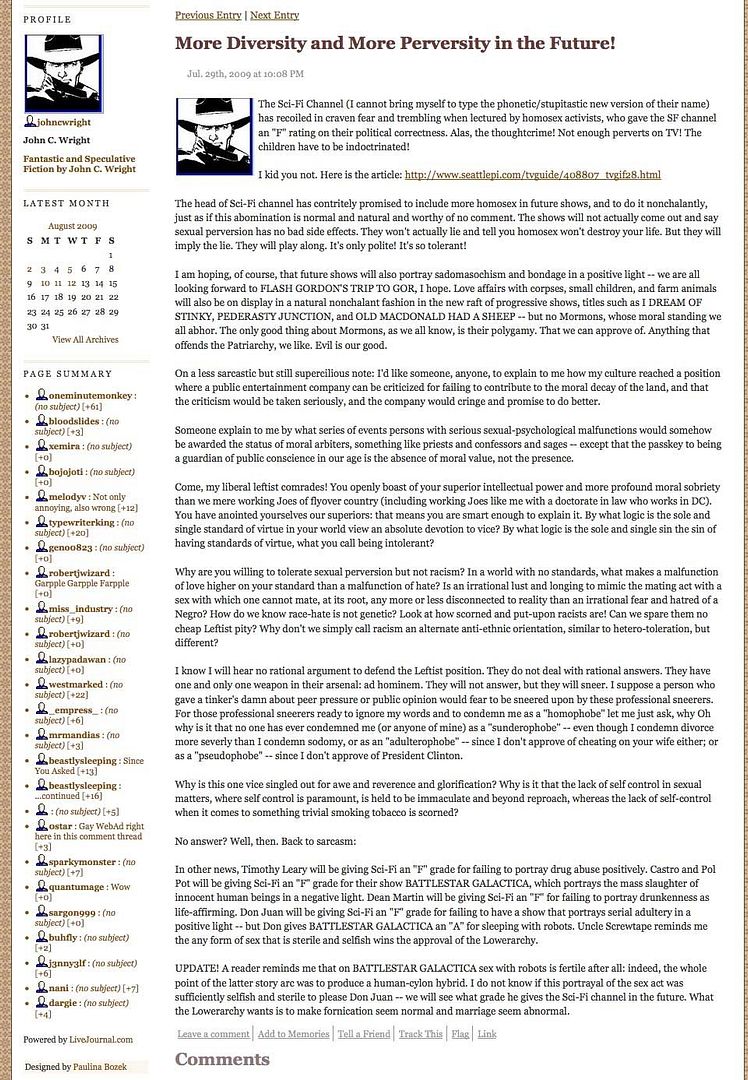The webpage described is cluttered with dense text and appears to have been poorly printed, likely due to a malfunctioning printer that resulted in some parts of the text being more legible than others. The central image on the page features a man dressed as a classic outlaw or cowboy, donning a cowboy hat and a bandana partially covering his face. This figure, reminiscent of an old-fashioned detective or a menacing character, is identified as John C. Wright. Beneath the image, the page title "Previous Entry" and "Next Entry" are displayed.

On the left side, there is a navigation menu containing various sections such as "Profile," "Fantastic and Speculative Fiction by John C. Wright," "Latest Month: August 2009," "Archive," "Page Summary," and a variety of user names or participant links. 

The main content in the center begins with a title "More Diversity and More Perversity in the Future," dated July 29th, 2009, from 10 am to 8 pm. The article criticizes the Sci-Fi Channel for its attempts to increase representation of homosexual characters under pressure from activists, conveying strong sarcasm and disapproval. The text includes a link to an external article, followed by sections of text printed with varying quality, reflecting possible printer issues.

The content is highly opinionated, discussing the perceived impact of increased sexual representation on television, with numerous sarcastic remarks about political correctness and social tolerance. The article concludes with options for interaction including "Leave a comment," "Add to Memories," "Tell a Friend," "Track This," and "Flag or Link," yet no comments are visible.

Overall, the page is a blend of fervent opinion, social commentary, and technical presentation issues.